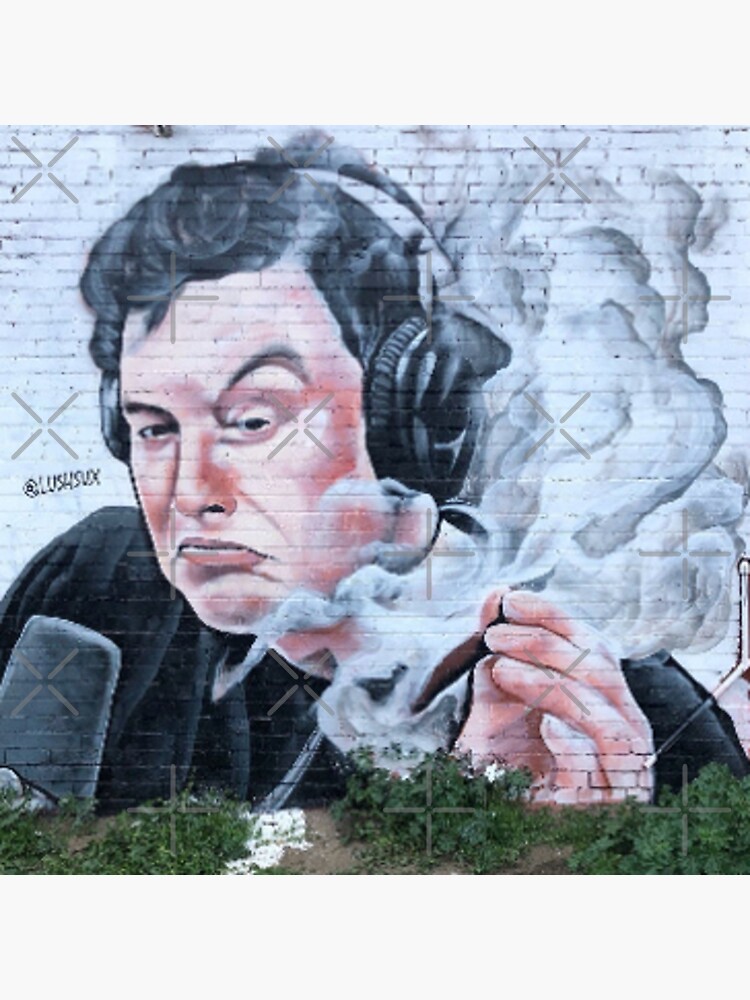The image captures a detailed photograph of a vibrant graffiti mural, set against a cream-colored brick wall background. In the foreground, scraggly plants and bushes partially obscure the base of the building. The mural, which spans a significant portion of the wall, portrays a stylized depiction of Elon Musk. He is wearing thick black headphones, connected by a silver strap, and has a microphone positioned in front of him. Musk's expression is notable, with his left eyebrow raised and his mouth slightly strained in a "look what I'm doing" kind of face, as he smokes a blunt, evidenced by the swirling smoke around his face. The mural artist has tagged the piece with "Lush Sux" in the bottom left corner. A transparent gray watermark of intersecting X and plus symbols overlays the entire image, adding a subtle but noticeable layer to the photograph.